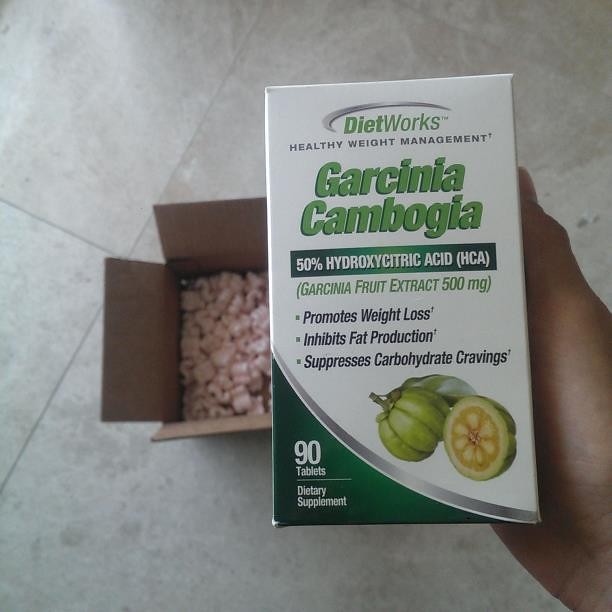This image depicts a bottle of Garcinia Cambogia dietary supplement from the brand DietWorks. The supplement is designed to support healthy weight management and prominently features 50% Hydroxycitric Acid (HCA), derived from Garcinia fruit extract at a concentration of 500 milligrams. The product is marketed to promote weight loss, inhibit fat production, and suppress carbohydrate cravings. 

At the bottom left corner, the label clearly states "90 tablets" in white lettering against a dark green background, indicating the quantity of the dietary supplement. The image also shows a Garcinia fruit, which is green on the outside with a yellow interior, encircled by a mix of green and white colors. The bottle appears to be displayed in an open box, surrounded by packing peanuts, suggesting it has recently been unboxed.